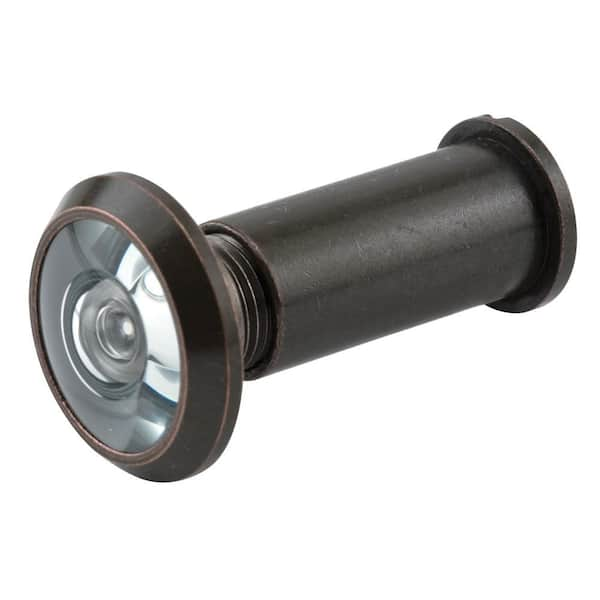This photograph depicts a cylindrical light fixture positioned against a completely white, featureless background, often used for commercial settings such as online shops, listings, or catalogs. The fixture, resembling a unique and creative flashlight, lies horizontally in the square-shaped image. The larger rounded disc, which has a glass lens-like quality and a dark grey to copper color gradient, is slightly screwed on the left side, while the smaller rounded disc points towards the upper right. Both ends feature glass elements suggesting illumination capabilities. The fixture itself appears industrial with a bronze-like texture and a beveled lip on the handle end. The photograph focuses on the object, providing no context for size or usage, emphasizing the product's details in an isolated, pristine backdrop.